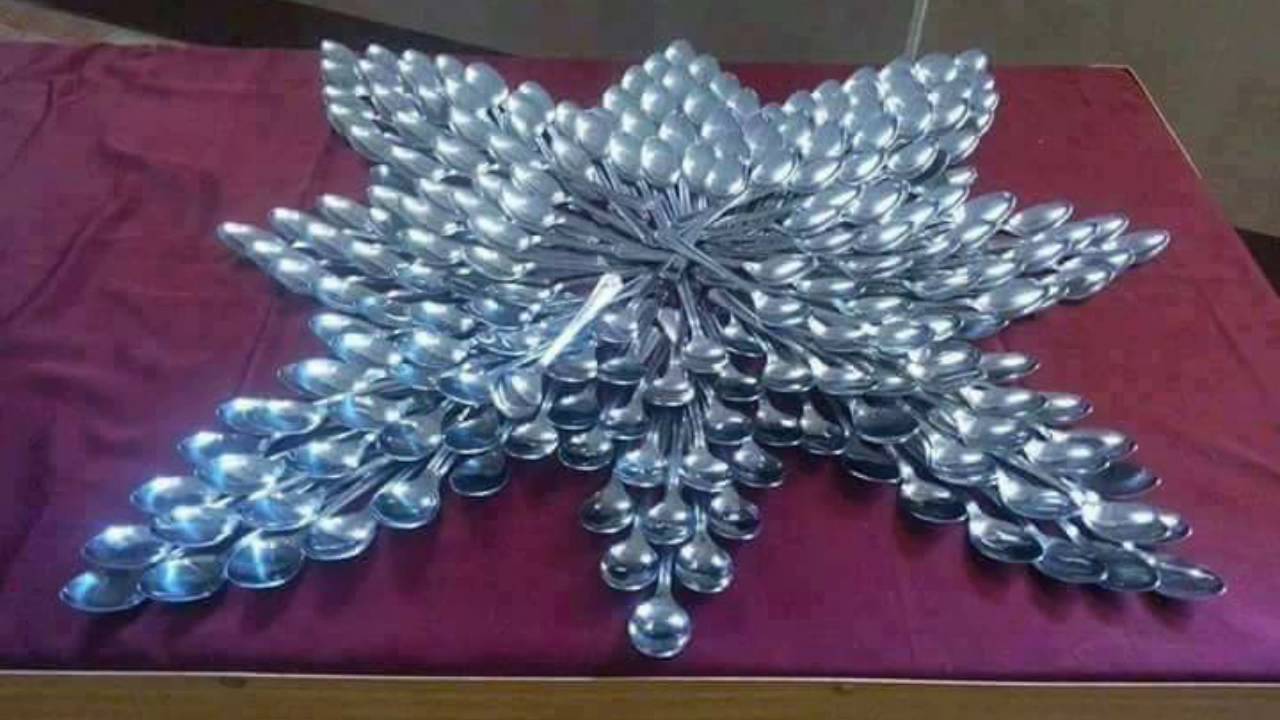The image showcases an intricate sculpture composed entirely of silver-colored stainless steel spoons, meticulously arranged to form an eight-point star or floral pattern. Each spoon is positioned with its head converging at the center, creating a symmetrical and striking visual effect reminiscent of a star or snowflake. This unique artwork is displayed on top of a dark maroon or red cloth, which rests on a brown platform, contrasting beautifully with the metallic sheen of the spoons. The background features a blend of brown and yellow tones, enhancing the composition, although the image appears slightly blurry.